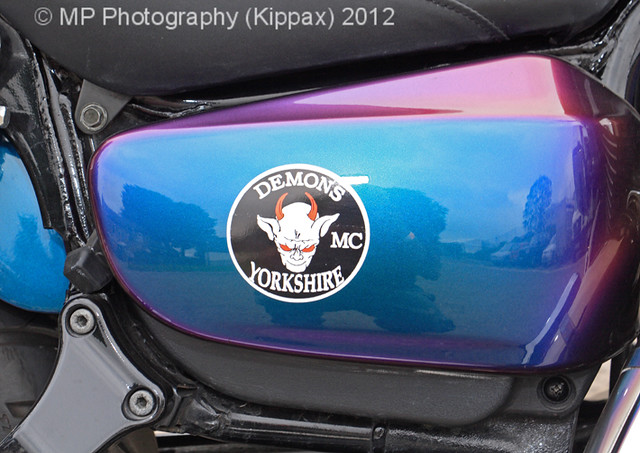The photograph captures a close-up of the metallic blue gas tank on a motorcycle, outlined with purple edges that give a burnt appearance. Prominently visible on the gas tank is a black circle with a white border, featuring the text "Demons MC Yorkshire" in bold white lettering. At the center of the logo, a white goblin-like creature with red eyes and inward-curving red horns stares out menacingly. Reflected on the shiny surface of the gas tank, one can discern the faint image of the photographer and a backdrop of cloudy skies and trees. The top portion of the photograph reveals part of a black leather saddle seat. Imposed in white font at the uppermost part of the image are the words "MP Photography, Kipax 2012," adding a touch of authenticity to this detailed and intricate capture.